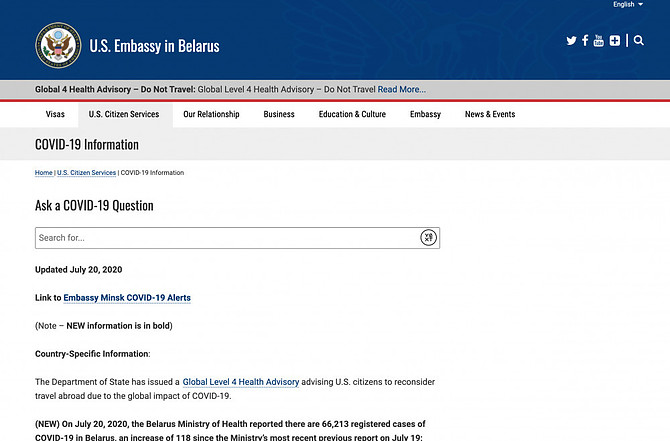This is a detailed caption for an image of a web page from the U.S. Embassy in Belarus:

---

The web page of the U.S. Embassy in Belarus prominently features the U.S. Embassy's symbol and the country's emblem at the top, framed by a navy blue stripe. On the right side of the stripe are icons for Twitter and Facebook, along with a plus image and a clickable search function. Beneath this, a light gray section announces a Global Level 4 Health Advisory with the text "Do Not Travel" followed by a "Read More" link.

Immediately below, a red bar delineates various sections of the website, such as Visa, U.S. Citizen Services, Our Relationship, Business, Education and Culture, Embassy, and News and Events. Further down, a gray bar provides updates on COVID-19 information and options to click for Home or U.S. Citizen Services, along with a searchable field to ask COVID-19-related questions. The page is updated as of July 20, 2020.

A link leads to Embassy updates titled "EMBASSY MINSK COVID-19 Alerts," where critical updates are emphasized in bold text. The country-specific information indicates that the U.S. Department of State has issued a Global Level 4 Health Advisory, advising U.S. citizens to reconsider international travel due to the global impact of COVID-19.

In bold at the bottom, the page notes that as of July 20, 2020, the Belarus Ministry of Health reported 66,213 registered cases of COVID-19, reflecting an increase of 118 cases since the previous day's report on July 19. The page stresses the importance of timely updates and includes links for detailed forecasts and documentation on recent information and state-specific advisories.

---